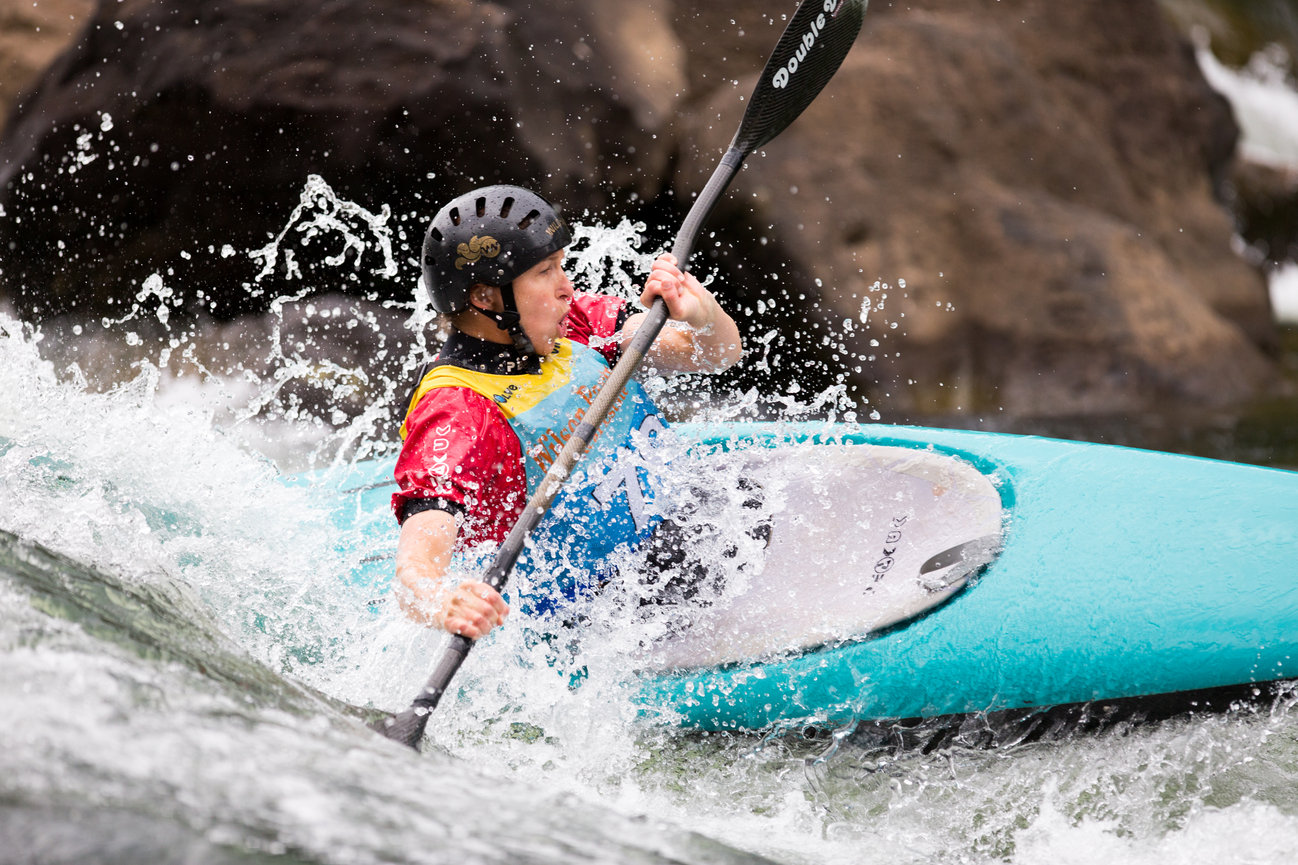In this dynamic daytime photograph, a single person is captured whitewater kayaking down a rough section of water, with splashes of white rapids all around. The vibrant aqua blue kayak, detailed with a white oval center where the kayaker sits, stands out against the tumultuous water. The kayaker, a Caucasian man, is wearing a multicolored safety vest featuring shades of yellow, light blue, and dark blue, over a vivid red short-sleeve wetsuit. To ensure safety, he dons a black helmet adorned with gold imagery and holds a gray double-sided paddle, which has the word "double" written in white. The image highlights the intense motion as one end of the paddle dips into the water while the other stands upright, reflecting the rower's fast-paced action. Behind him, towering and jagged deep brown cliffs form a dramatic backdrop, slightly out of focus due to the intensity of the rapid movement in the foreground. The photograph encapsulates the thrill and danger of whitewater kayaking against a rugged natural setting.